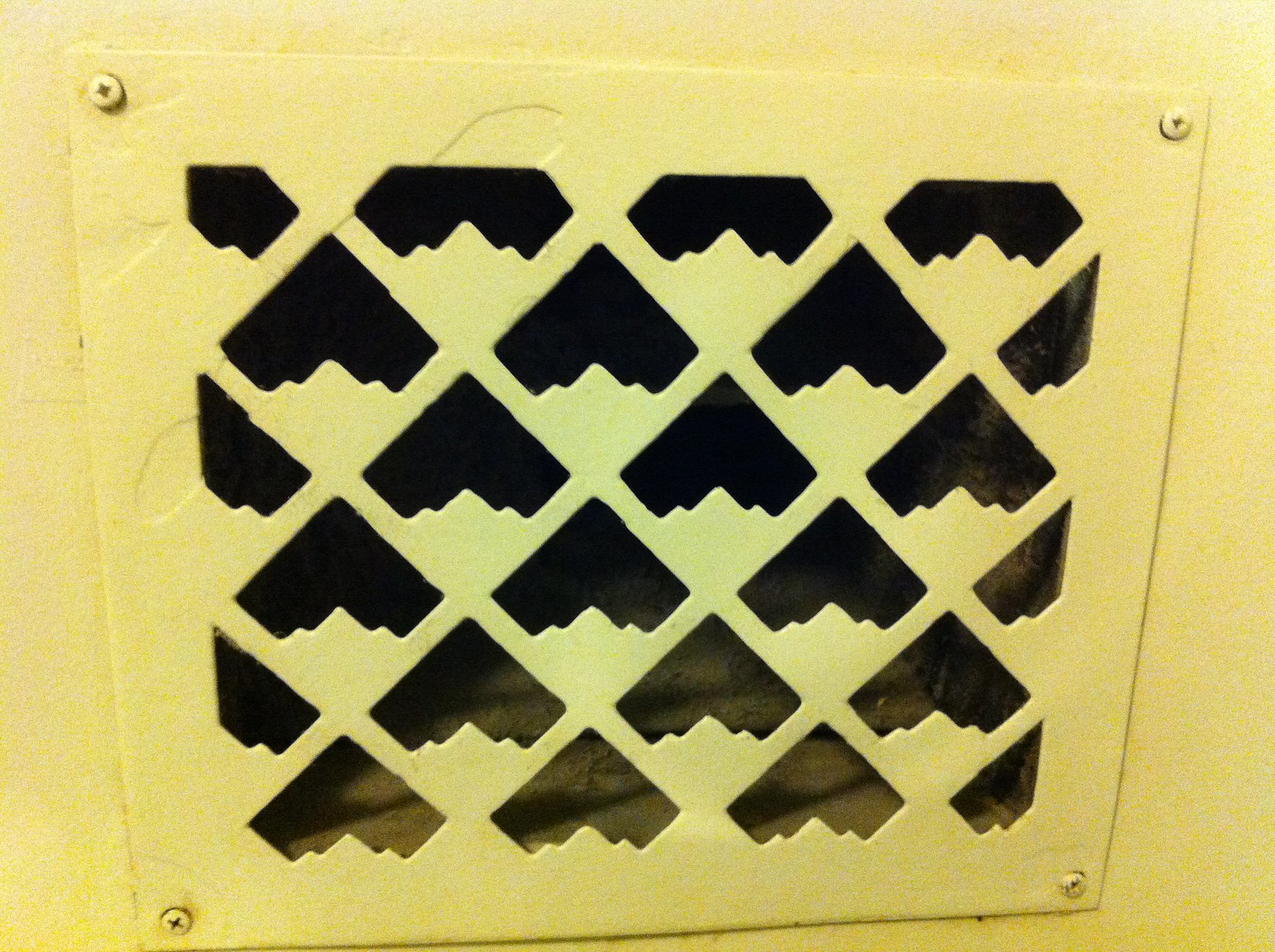This image features a close-up of a uniquely designed yellow vent panel mounted on a matching yellow wall. The panel is secured by four yellow-painted screws, one in each corner. The vent openings are cut into symmetrical, arrow-like geometric patterns, somewhat reminiscent of a stealth bomber's shape with triangular points and boxy edges. The bright yellow paint uniformly covers the wall, panel, and even extends inside the vent, although the interior is mostly dark and appears slightly dirty. The precision of the pattern and the uniformity of the yellow paint, despite some minor chipping and overspray, make this vent panel a striking and coherent visual element against the yellow backdrop.